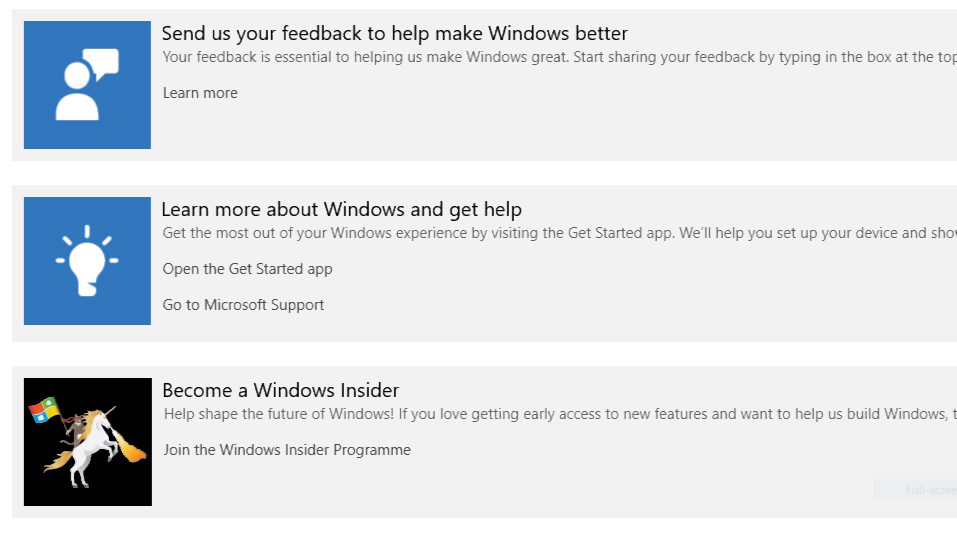This image is a cropped screenshot taken from a computer, showcasing three distinct horizontal grey boxes with a small amount of white space separating each one. 

The first grey box features a blue square on the left side, containing an icon of a white person with a speech bubble above their head. Accompanying this icon is bold black text that reads, "Send us your feedback to make Windows better."

The second grey box also includes a blue square on the left, but this time the icon depicts a white lightbulb. Adjacent to this icon, bold black text states, "Learn more about Windows and get help."

The third and final grey box has a unique square icon on the left with a black background. The icon illustrates a person riding a white horse while holding a flag adorned with the Windows Microsoft logo. The text in bold black letters next to this icon reads, "Become a Windows Insider."